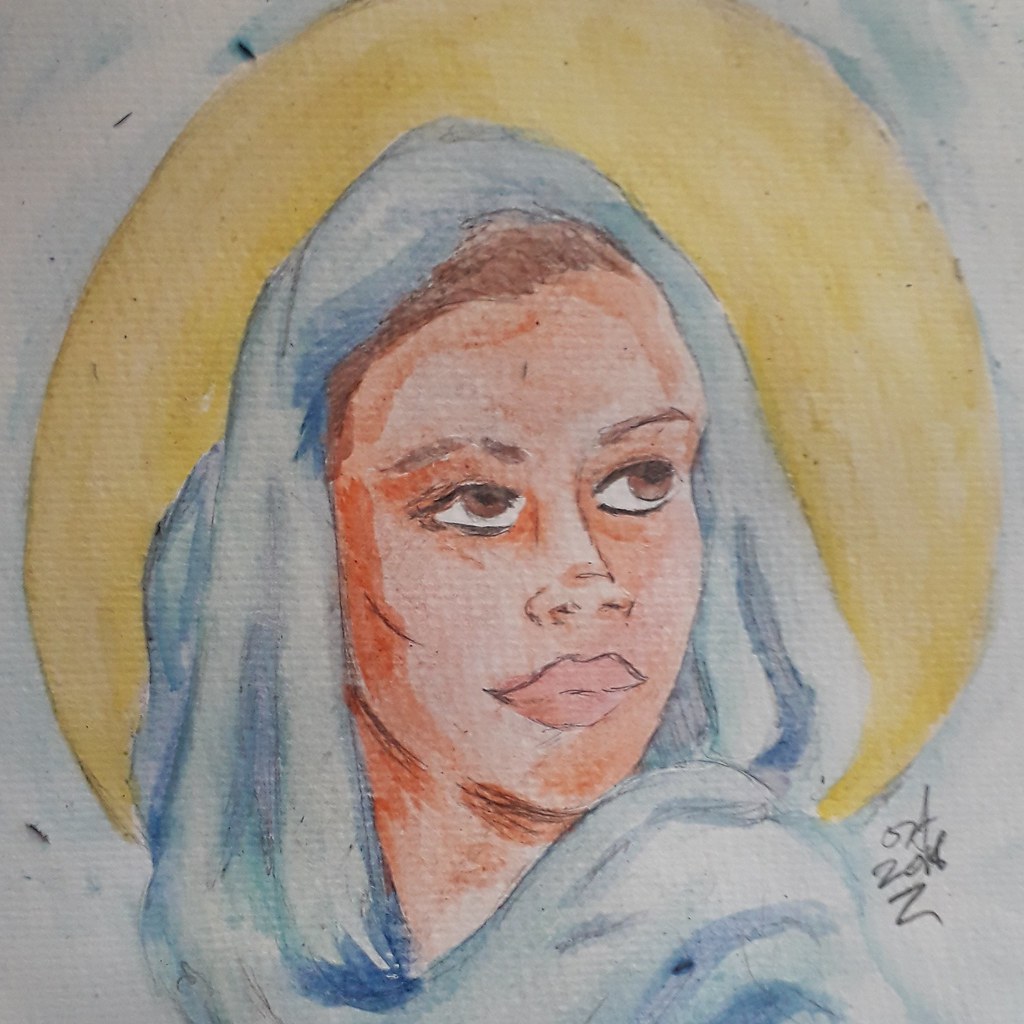This detailed watercolor drawing portrays a woman with an ethereal aura, reminiscent of the Virgin Mary. The subject has a serene expression, looking off to the side and slightly upward. She is depicted with brown eyes, brown hair, well-defined brown eyebrows, and full, voluptuous lips. Her head is adorned with a blue scarf or shroud that drapes over her shoulders and across her chest, suggesting modesty and grace. Behind her head, a radiant yellow halo signifies her sanctity, set against a background that blends white and shades of blue. The woman’s tan skin adds warmth to her portrayal, and her slight, confident grin enhances her captivating presence. The artwork is signed in black at the bottom right corner, appearing as two Z's, possibly indicative of the artist's initials or signature from 2018.